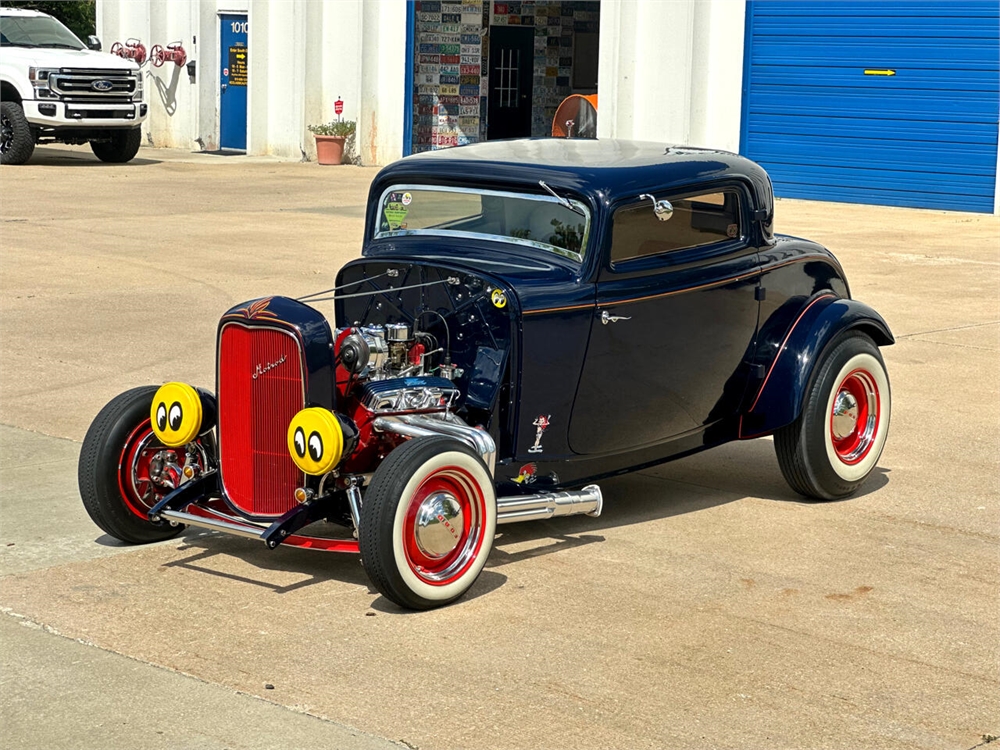The photograph captures a vintage '32 Roadster hot rod parked prominently in the foreground on a concrete driveway in front of a mechanic's shop with two garage doors—one open and one closed. The Roadster, possibly a modified Model A Ford, boasts a sleek black body and a hardtop roof, emphasizing its classic yet aggressive stance. Its large round headlights are adorned with yellow caps, topped by playful white and black googly-eyes, enhancing its distinctive character. The car features a striking red grille and exposed engine detailing, revealing chrome exhaust pipes and fire-red valves, indicating its high-performance V8 setup. The rims are also painted a vibrant red, paired with wide whitewall tires, adding to its vintage charm. To the left in the background, there is a large Ford F-350 pickup truck parked, contributing to the automotive atmosphere of the scene.